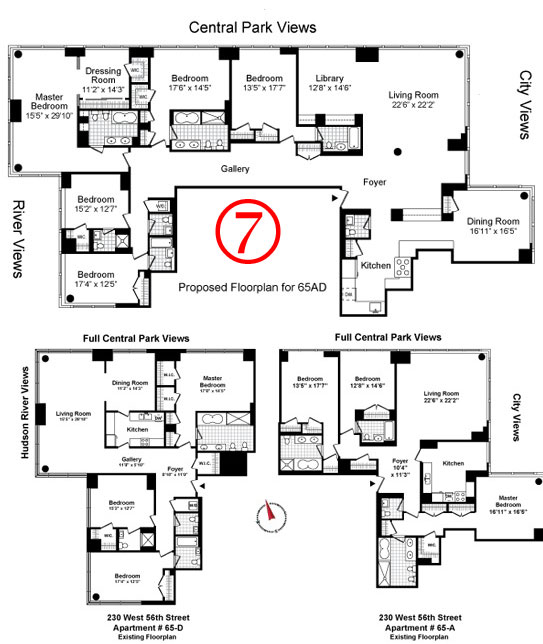This detailed caption accompanies a photograph depicting an apartment complex layout with various floor plan options. The diagram, rendered in black ink on white paper, showcases three distinct floor plan designs. The top section of the diagram highlights apartments with Central Park views, while the right side indicates City Views, and the left side is marked with River Views, specifically Hudson River Views. Each floor plan is intricately detailed, with the top option featuring four bedrooms and a master bedroom, and the two smaller layouts comprising two bedrooms and a master bedroom each. A striking feature is the red circled number 7 situated centrally within all three plans. Additionally, a gray circle with an outwardly protruding red arrow or dial is positioned at the bottom between the two smaller floor plans, though it lacks a specific label.